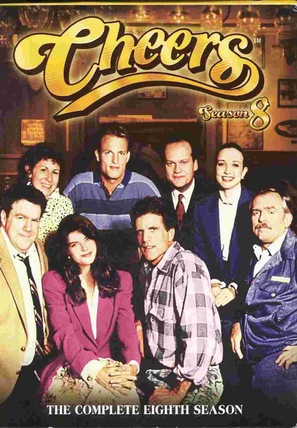This is a cover for the DVD of the television series *Cheers: The Complete Eighth Season*. The vintage-style poster showcases the iconic bar setting in the background with its amber-gold hues and vintage architectural elements like the grand brown walls and multiple ornate lights. At the top, the title *Cheers* is prominently displayed in golden fonts, followed by "Season 8". The bottom features the tagline "The Complete 8th Season."

In the forefront, the main cast is arranged with a mix of standing and seated poses. Centered is Kirstie Alley, with long black hair and dressed in a red vest and skirt. To her right sits Ted Danson, sporting a white and black plaid shirt. To Kirstie’s left is the character Norm, wearing a yellow suit, brown tie, and white shirt, distinguished by his short black hair. Behind Norm stands Carla, in a floral shirt, smiling. Ted Danson's character is flanked by others, including Woody Harrelson in a light and dark blue striped shirt, and Frasier, dressed in a black suit with a red tie. Frasier's serious-looking wife, also smiling, is in a matching suit with her black hair pulled back.

Additional cast members fit the setting: a man in a shiny blue jacket and another in a brown jacket. Lastly, the mailman character, dressed in his blue uniform and sporting a mustache, appears at the bottom right. The ensemble cast exudes the charm and camaraderie of the beloved series, captured in full color, with their warm smiles and iconic wardrobes vividly standing out.